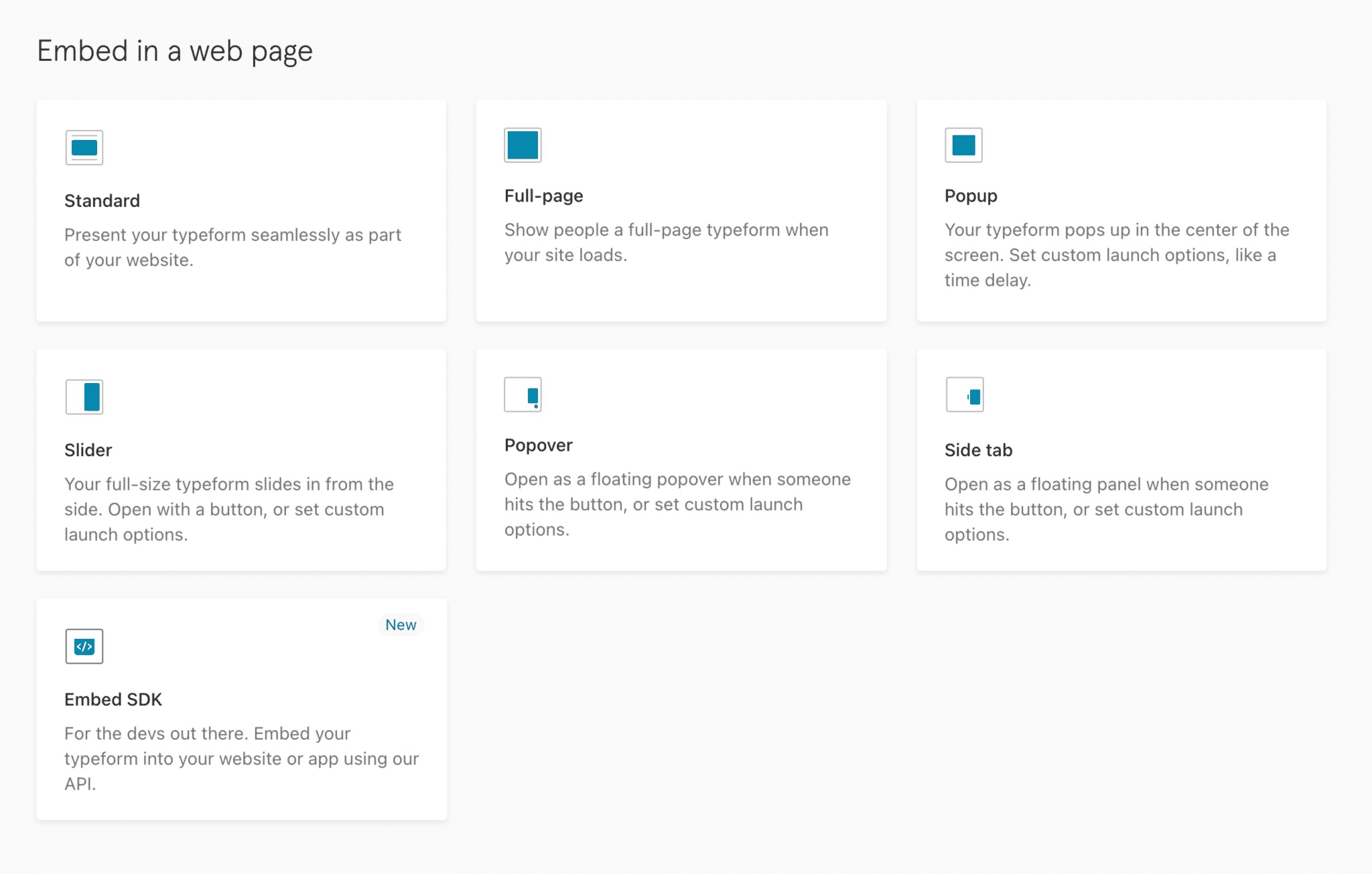The image showcases a set of guidelines for embedding Typeform into a webpage, organized into seven distinct methods, each represented by a box containing text and an icon or logo. Here's a detailed descriptive caption:

---

**Embedding Typeform into Your Webpage: A Visual Guide**

At the top of the image, a header reads "Instructions to Embed Typeform into Your Webpage." Below this header, there are seven boxes arranged from left to right, each illustrating a different method for integrating Typeform into a website.

1. **Standard Embed**: The top-left box describes how to present your Typeform seamlessly as part of your website. This is a straightforward embedding method to make the form look native to your page.

2. **Full Page**: Appearing next, this box explains how to display a full-page Typeform that loads as the entire page view when your site is accessed.

3. **Pop-up**: The middle-left box features an image of a form popping up in the center of the screen, with text explaining that the Typeform can appear as a pop-up with customizable launch options such as a time delay.

4. **Slider**: Located next, this box shows a Typeform sliding in from the side of the page. It can be triggered by a button or custom launch settings, and takes up a full section of the screen.

5. **Popover**: This box depicts a floating popover form that appears when a user clicks a button, with additional text detailing how to set custom launch options.

6. **Side Tab**: To the right is a box showcasing a floating panel Typeform that opens when a button is clicked, again with options for custom launches.

7. **Embed SDK**: The final box at the top-right is labeled "NEW" and is geared towards developers, indicated by the text "For the devs out there." It describes embedding the Typeform into a website or app using an API.

These options provide various ways to integrate engaging forms into your site, enhancing user interaction tailored to different design and functionality needs.

---